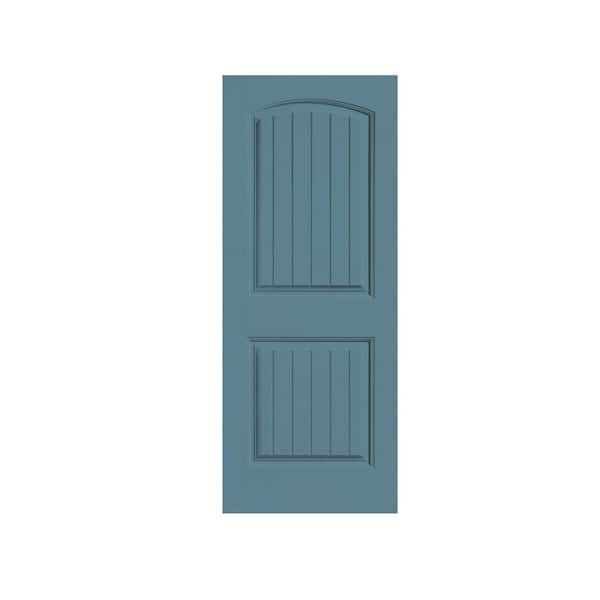The image depicts a blue door set against a stark white background. The door, which is taller than it is wide, has a rectangular shape with distinct architectural details. The top section of the door features an arched rectangle with multiple thin, embossed wooden slats running vertically inside it. Below, there's a square panel, also filled with thin, rectangular slats, adding texture to the design. The door's color might be described as either a dark teal, light blue, or bluish-gray, highlighting its textured and embossed wooden pattern. This combination of detailed indentations and slats creates a unique visual element on the plainly colored, rectangular door.